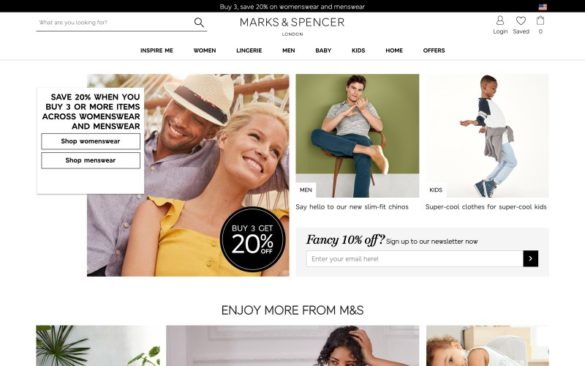This is a screenshot of the homepage for Marks & Spencer London, a prominent clothing company. At the very top of the screen, a black banner features a promotional offer in white text: "Buy 3 Save 20% on womenswear and menswear." To the left of the central company logo, a search bar is available, labeled "What are you looking for". To the right of the logo, there are clickable options for "Login," "Saved," and the "Shopping Bag."

The primary navigation menu is positioned below the logo, featuring categories in the following order: Inspire Me, Women, Lingerie, Men, Baby, Kids, Home, and Offer. Beneath the navigation, the main content area displays a collage of six diverse images. These include:
1. A man and a woman smiling.
2. A man sitting casually in a chair.
3. A child standing on their toes.
4. A very young child lying on their side.
5. A woman sitting pensively with her hand resting on her head.
6. A partial image of an array of plants.

Additionally, there is a prominent text box showcasing the offer to "save 20% when you buy three or more items across womenswear and menswear," accompanied by two clickable buttons labeled "Shop Womenswear" and "Shop Menswear."

Towards the bottom, there is an area for visitors to enter their email addresses to sign up for the company's newsletter, with the added incentive of receiving 10% off their order.